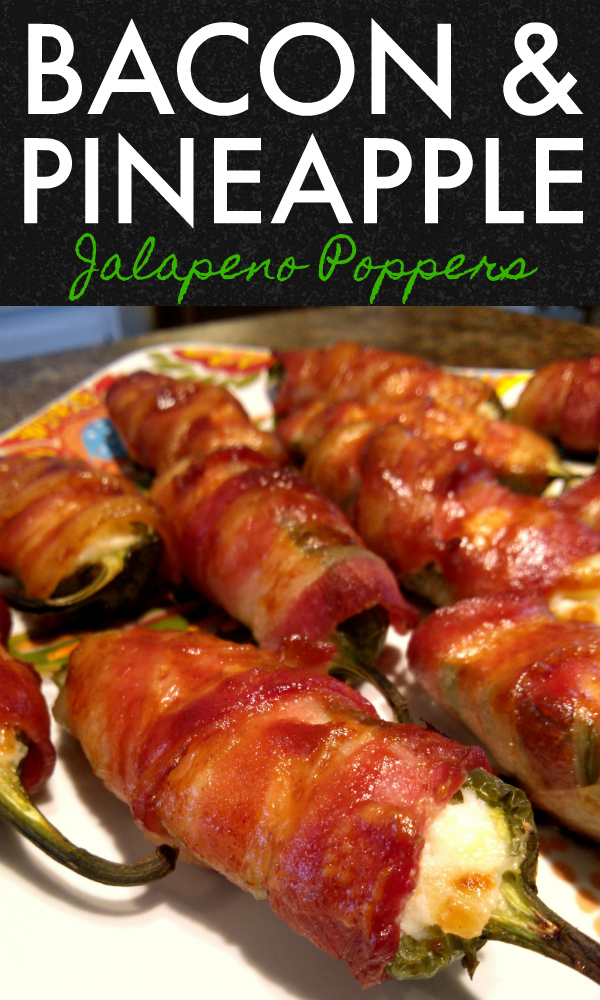The image is a vertically aligned rectangular photograph that resembles a recipe book cover or a restaurant sign. The top third of the image features a solid black background with bold white text that reads "BACON AND PINEAPPLE" in all caps. Below this, in green cursive, it says "JALAPENO POPPERS." The lower portion of the image showcases several jalapeno poppers arranged on a white plate with a yellow and red patterned design, which sits on a brown table or countertop.

The jalapeno poppers are wrapped in crispy bacon and are visibly stuffed with pineapple and cheese, with some cheese oozing out, giving them a glossy, well-cooked appearance. There are about six to eight poppers in the image, with the foreground popper displaying a crusted exterior with tones of brown and orange and a hint of green from the stems. The poppers appear slightly blurred as they recede into the background, adding depth to the composition.